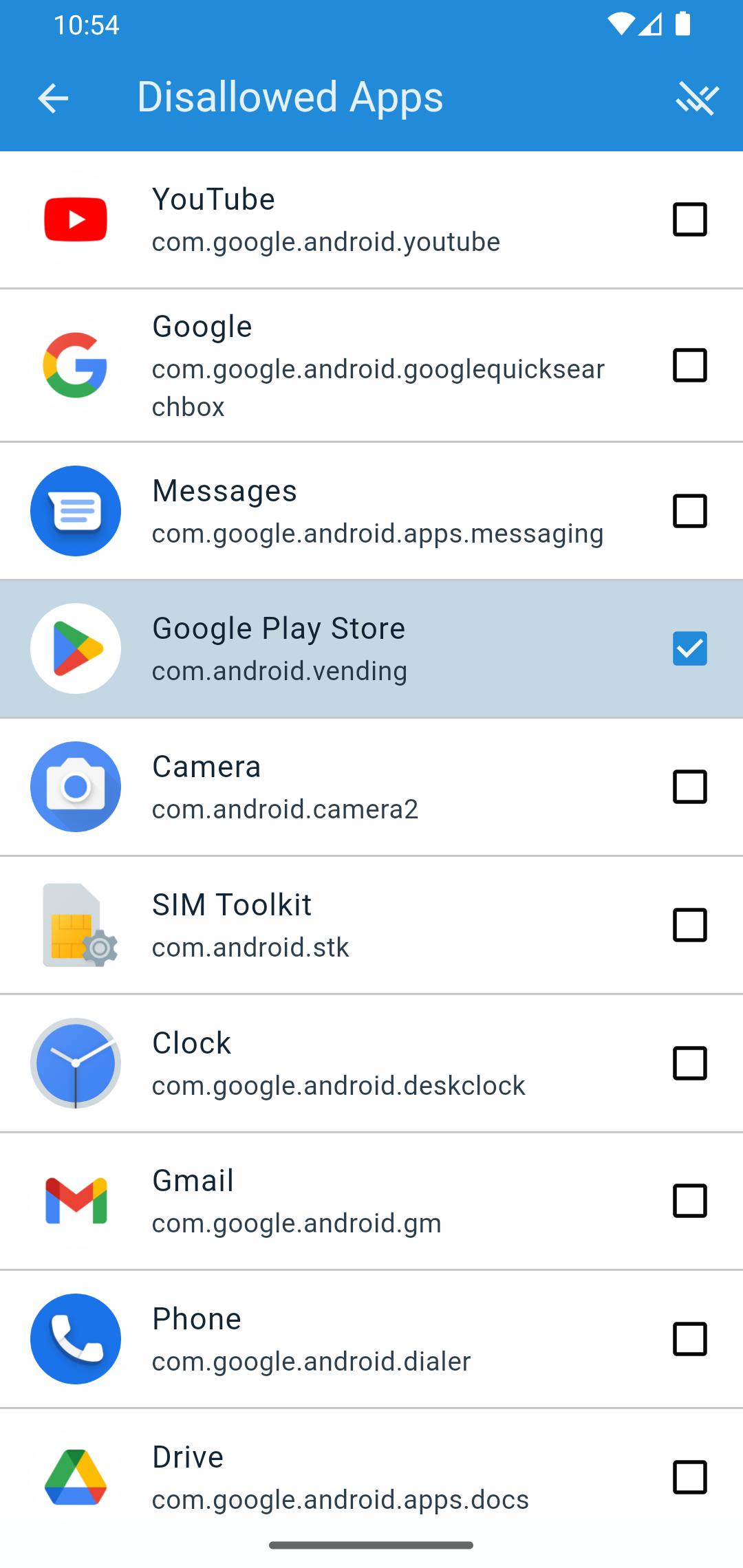The image displays a smartphone screenshot with a blue border at the top, indicating the current time as 10:54. It shows a Wi-Fi signal strength of 2 out of 4 bars and a partially filled battery icon. Below the status bar, there is a left-pointing arrow labeled "Disallowed Apps."

The main portion of the screen has a white background, listing applications with their respective icons on the left and checkboxes on the right. Each entry includes the app name and its internal package name, framed by a light gray border. The listed apps are:

1. YouTube - youtube.com.google.android.youtube
2. Google - google.com.google.android.googlequicksearchbox
3. Messages - messages.com.google.android.apps.messaging
4. Google Play Store - com.android.vending (This app has a blue checkbox with a white checkmark indicating it is selected)
5. Camera - camera.com.android.camera2